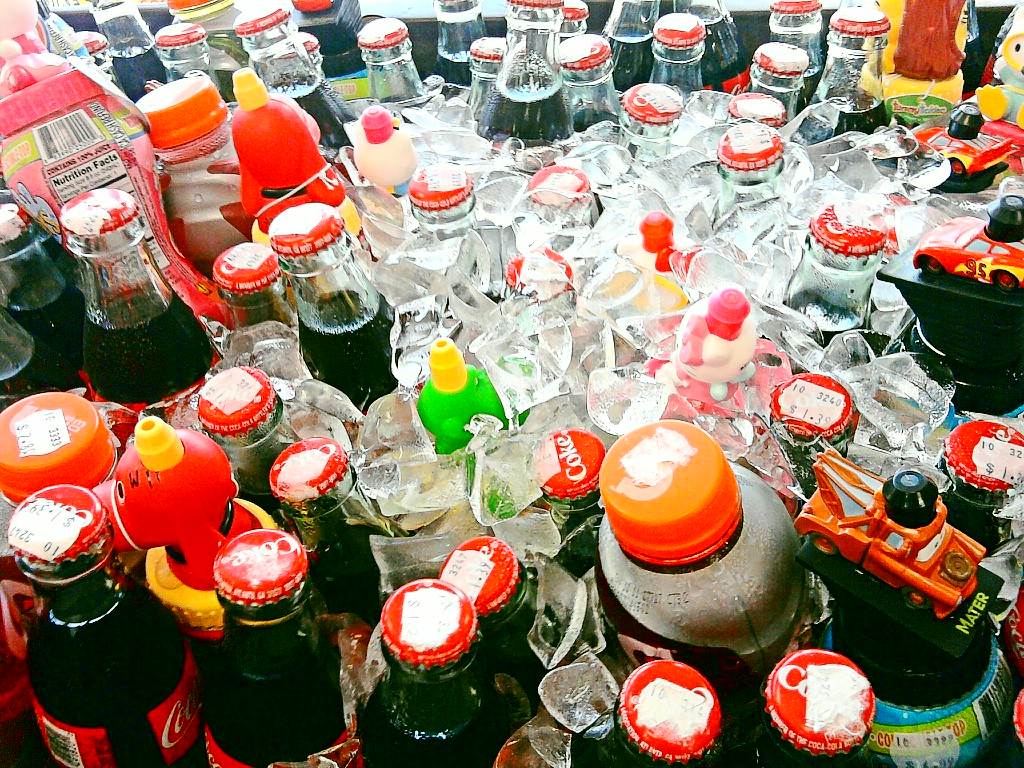This vibrant, color photograph prominently features a sprawling collection of Coca-Cola glass bottles, each filled with the iconic dark liquid and topped with traditional twist-off red metal caps. Some of these caps reveal the classic white curly "C" and the start of "O". These bottles are densely packed and extend all the way to the back of the image, with their labels partially obscured by a generous scattering of clear ice cubes—most resembling the type produced by commercial ice machines, appearing as imperfect squares and rectangles.

Among this sea of Coca-Cola bottles, a variety of other drinks can be noted. These include plastic bottles of differing shapes, some with pink labels and others featuring silver labels paired with orange tops. Additionally, there are sporadic appearances of green bottles with yellow tops and red bottles also capped with yellow tops.

Interspersed throughout the image are whimsical elements such as toy cars. One prominent toy car in the foreground is an orange tow truck. Nearby, another toy car is red with yellow details, marked with the number "95". Positioned near the top right, we notice a yellow-skinned toy wearing a light blue shirt and shorts, distinctive with its big yellow feet.

All these elements combine to create a dense, detailed tableau dominated by Coca-Cola and punctuated with a mix of other beverages and playful toys, making it a lively and engaging scene.